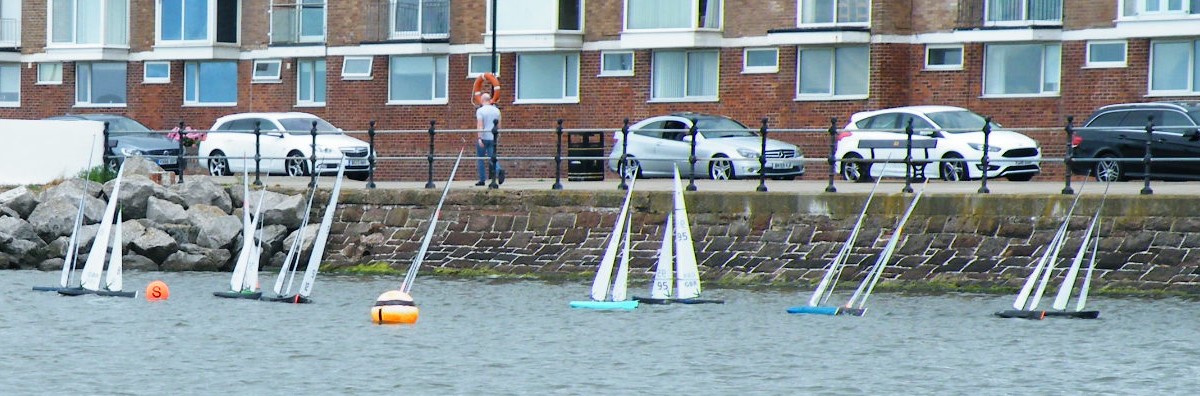This color photograph, taken outdoors on a sunny day, captures a tranquil scene by the water, likely a small river or lake. The body of water is calm and clear, hosting twelve small remote-controlled sailboats with long white masts and various colored hulls, including black, blue, navy blue, and olive green. These sailboats appear to be engaged in a race or a leisurely float, accentuated by a couple of buoys—one yellow and one orange—floating around them.

In the background, a slightly elevated embankment leads to a parallel street where several cars are parked. The lineup includes two white cars, a gray car, two black cars, and another unspecified vehicle. The street is bordered by a brick sidewalk, and beyond that, there's a two-story brick apartment building with numerous windows. Stacked gray stones and a metal fence run along the length of the embankment, reinforcing the idyllic charm of this picturesque urban waterfront.